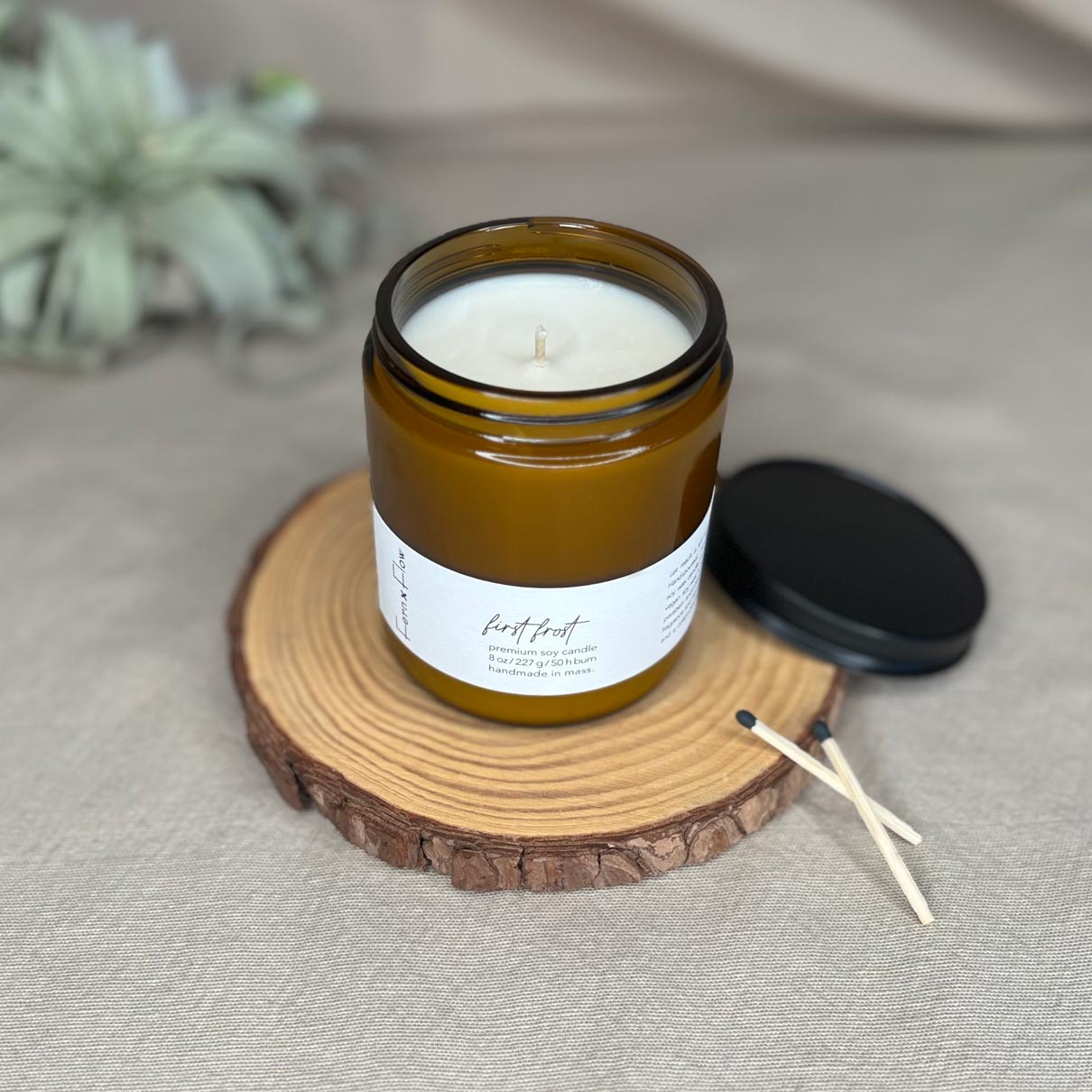In this image, a white candle is set inside a brownish-green glass jar with a white label near its base. The label, written in script font, reads "First Frost," accompanied by additional details in regular font: "Premium Soy Candle, 8 ounces (227 grams), 50 hours burn, Handmade in Mass." The black lid of the jar is placed to the side, revealing the white candle and its centered white wick. The jar and its lid rest on a slice of a tree trunk, showcasing visible concentric rings and rough bark edges, giving it a rustic look. Two used matches with black tips lean against this wooden coaster. The scene is set against a white or gray linen backdrop, adding a soft and neutral tone, while in the upper left corner, a green plant with large leaves provides a touch of natural greenery to the composition.